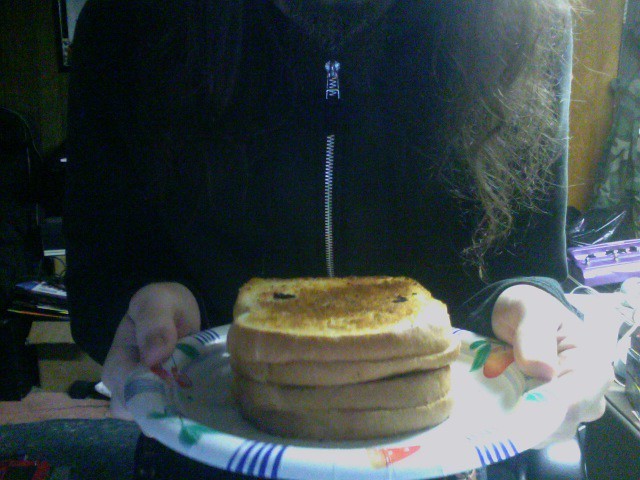This color photograph features a young woman holding a paper plate with four slightly well-toasted slices of bread stacked perfectly on top of each other. The focus of the image is on the plate of toast, which is held close to the camera with the woman's hands grasping either side. The toast appears to be white bread, with some pieces showing a light brown color and a few possible burnt spots or raisins.

The paper plate is white with blue stripes pointing inward and decorated with colorful fruit illustrations, including a pear and an apple. The woman is wearing a black, long-sleeve, zip-up hoodie with a silver zipper zipped all the way up. Her long, wavy brown hair, which is slightly frizzy, falls down in front of her shoulders, and her pale hands, with fingers underneath the plate and thumbs on top, hold it out in front of her chest.

The background is cluttered, featuring items such as a camo jacket hanging on a door, boxes piled on the floor, a purple object, and a black trash bag. There is a lot of light coming in from the right side of the photo, causing a glare that partially washes out some details and makes them blurry.